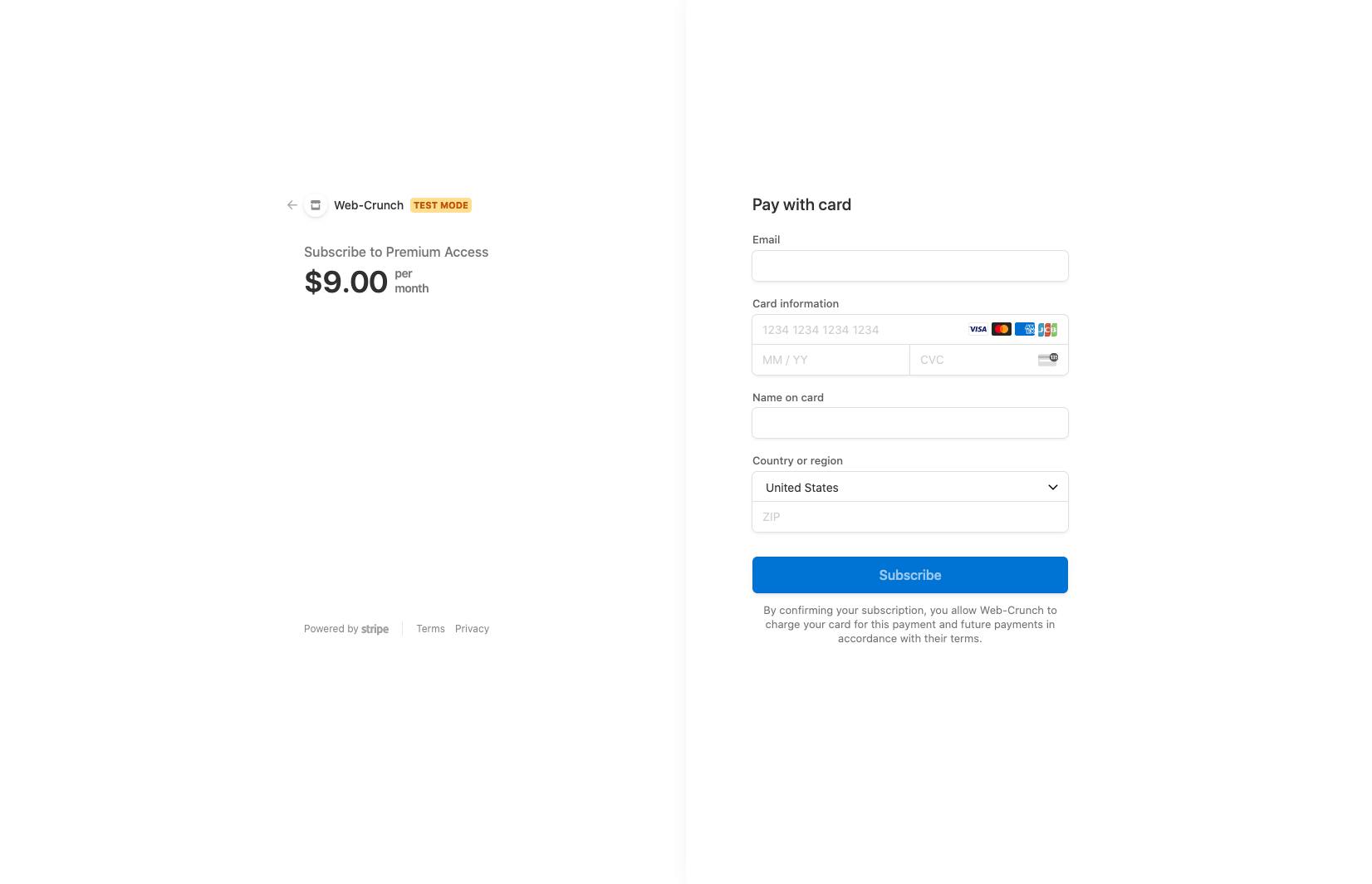The image depicts an order screen from a webpage. In the top left corner, in very small and hard-to-read letters, it says "Webcrench". Directly below this is an orange box that indicates "Test Mode". 

The main section of the page features a subscription offer: "Subscribe to Premium Access, $9 per month". The "$9" is prominently displayed in large, bold numbers, while the rest of the text is in a much smaller font.

At the bottom left of the image, there's some text that's difficult to decipher, but it includes clickable options for "Terms" and "Privacy".

On the right side of the screen, there is a form to enter payment details. It is titled "Pay with Card" and includes the following fields:

1. An email address field.
2. Three fields for card information: the card number, the expiration date, and the security code (found on the back of the card).
3. A field for the name on the card.
4. A field for the country of origin, which shows "United States" as the currently selected option.
5. A field for the zip code.

Below the form fields, there's a blue "Subscribe" button. Some additional text appears below the button, but it is too small to discern any details.